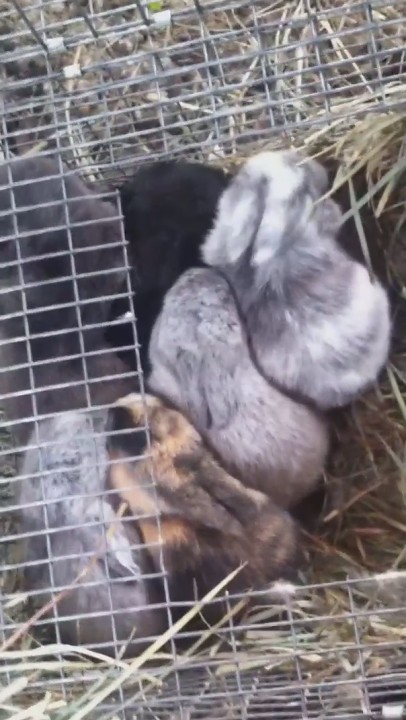The image appears to be a top-down view of six adult bunny rabbits huddled together in a pen, likely captured from a low-quality video or a low-resolution phone camera. The photograph, which is tall and thin, shows a pixelated scene with the bunnies confined in a small metal cage lined with straw at the bottom. The lighting is neutral, making it difficult to discern whether it is artificial or natural. The rabbits are varied in color; most are gray with some displaying white patches, while a black rabbit and a brown-and-black calico bunny can also be seen. The bunnies are nestled closely together, with a few partially obscured by the cage. Despite the blurry quality of the image, the rabbits' ears can be discerned pointing straight back. The cage appears to be resting on grass, and the top is open, giving an unobstructed view of the clustered animals.